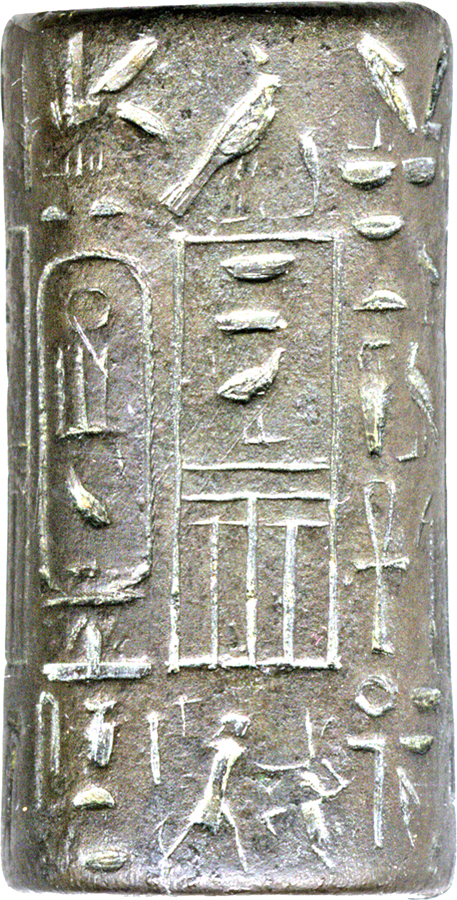The image features a rectangular ancient Egyptian stele, resembling a gravestone. Crafted from tan-grayish-green stone, the surface is intricately detailed with Middle Egyptian hieroglyphs, carved into the material and appearing in white or cream color. The stele is adorned with an array of symbols and images: birds, baskets, an ankh, tool, bowls, ribbons, and several human figures engaged in various tasks. The top part showcases images of a sun, sheaves of wheat, and a fish, while the left side displays a cartouche-like oblong rectangle with hieroglyphic characters, including a straight line with three equidistant vertical lines, a circle, and a fish-like symbol. The stone is weathered and aged, adding to its historic appeal. The bottom of the stele features a straight line crossed perpendicularly by another, with what appears to be a person holding an object beneath a large central rectangle, suggesting a significant narrative or inscription. Despite its age and wear, the stele's detailed carvings and symbols offer a glimpse into ancient Egyptian art and culture.